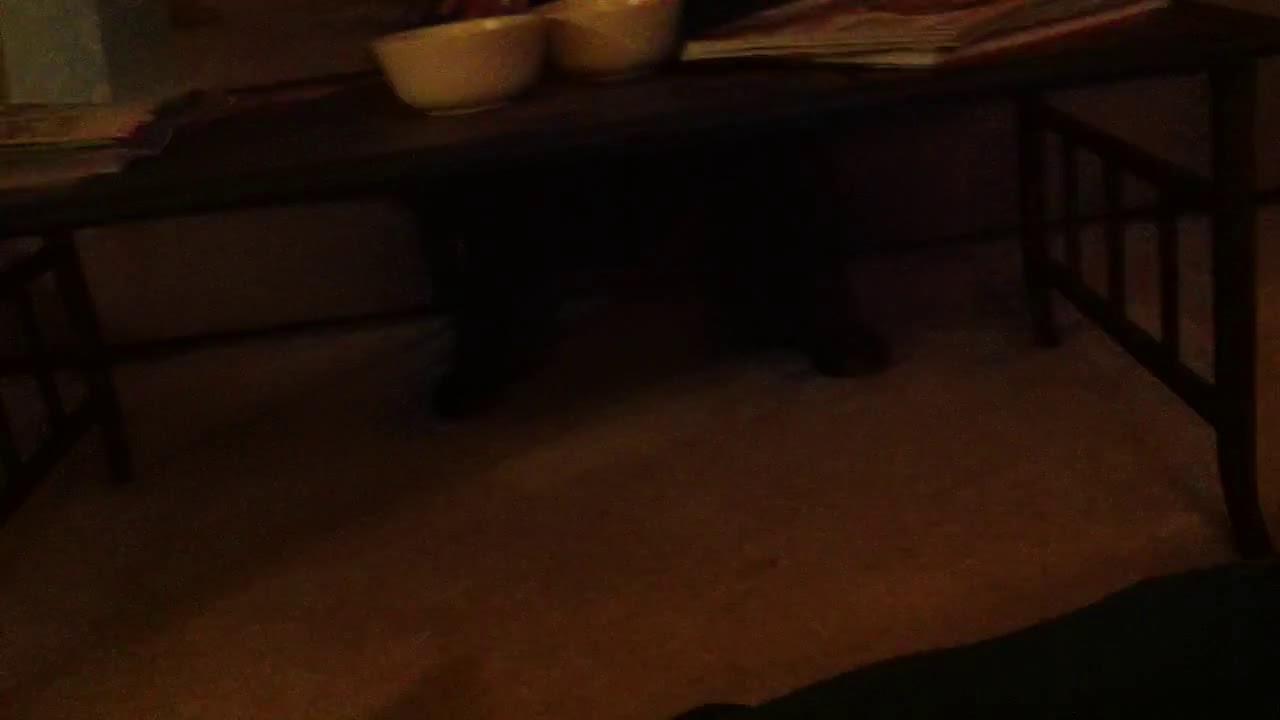The image depicts a dark and grainy photograph taken in low light, rendering it challenging to discern details clearly due to significant noise and compression. It features a small, low-to-the-ground, rectangular dark brown wooden table with a distinctive cross-section and bar-like framing on its legs, resembling fence sections. The table is set on what appears to be a white floor, possibly either a concrete or carpeted surface, indicating a dimly lit room with dark yellowish lighting. On the tabletop, two white ceramic bowls, akin to cereal or soup bowls, are placed centrally and adjacent to each other. Additionally, the table surface is cluttered with various items—a mix of books, magazines, and notepads along with possible pens or stationery, particularly concentrated on the right side. In the peripheral view, part of the wall with a green and white color scheme is visible in the top-left corner, contributing to the overall dark and compressed feel of the image.